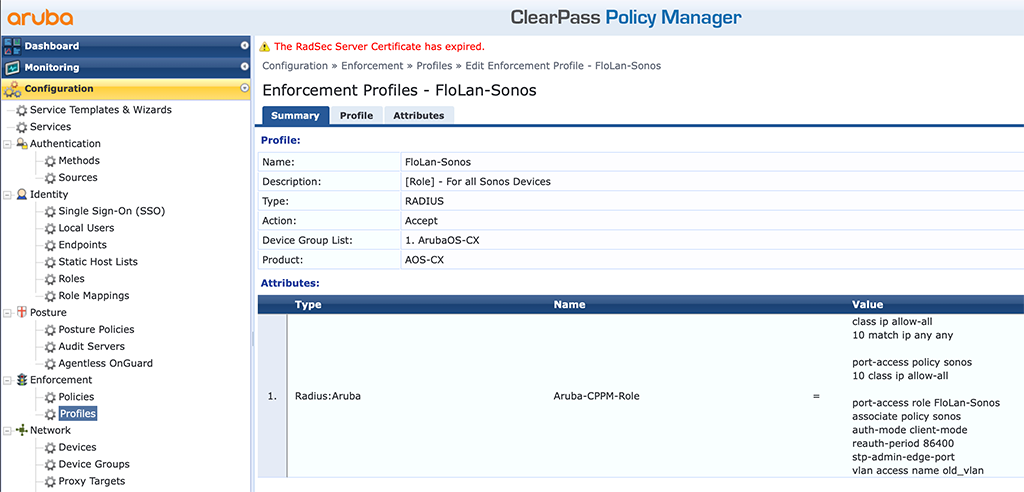In this rectangular image, a screenshot is presented against a white background, displaying a software interface. In the top left corner, a light gray banner is visible with the word "Aruba" printed in orange. To the right of this, the title "ClearPass Policy Manager" is shown. Below, an alert message in orange text reads, "The RADSEC server certificate has expired."

Further down in light gray text are multiple menu options: "Configuration," "Enforcement," "Profiles," and "Edit Enforcement Profile." Specifically, an enforcement profile named "FlowLAN Sonos" is being edited. The title "Enforcement Profiles" is displayed in black text, with "FlowLAN" and "Sonos" listed below, also in black.

Beneath these headings are three tab options. The currently selected tab, "Summary," is highlighted in dark blue, with white text. This summary tab displays detailed profile information, including:
- Profile name: "FlowLAN Sonos"
- Description: "Role for all Sonos devices"
- Type: "Radius"
- Action: "Accept"
- Device Group List: "1. Aruba OSCX"
- Product: "AOSCX"